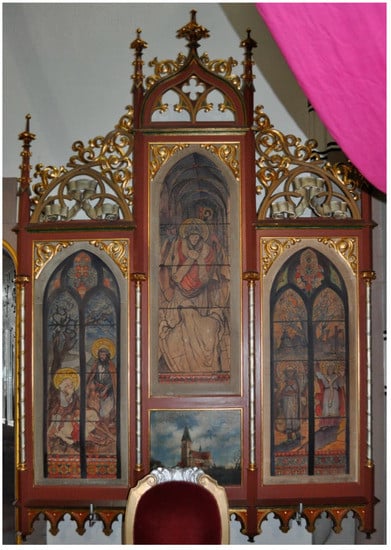In this photograph, there is an elaborate art piece prominently displayed in the center. The centerpiece is a wooden structure adorned with intricate golden designs that curl and wave towards the top, giving it an ornate and majestic appearance. Within this wooden frame, there are three individual sections that feature paintings designed to resemble stained glass windows. Each painting depicts a different scene: one shows two individuals tending to a lamb, another captures a person praying before another figure, and the third portrays two individuals standing beside a tree, all with halos of light around their heads, suggesting a religious or saintly context.

In front of this art installation, there's a stately gold wooden chair with an opulent red velvet seat, adding to the regal atmosphere of the scene. The background features stark white walls that contrast with the richness of the display, and a soft pink curtain intrudes from the upper right corner, providing a splash of color and a sense of elegance. The entire composition is meticulously detailed, creating a harmonious blend of artistry and craftsmanship.